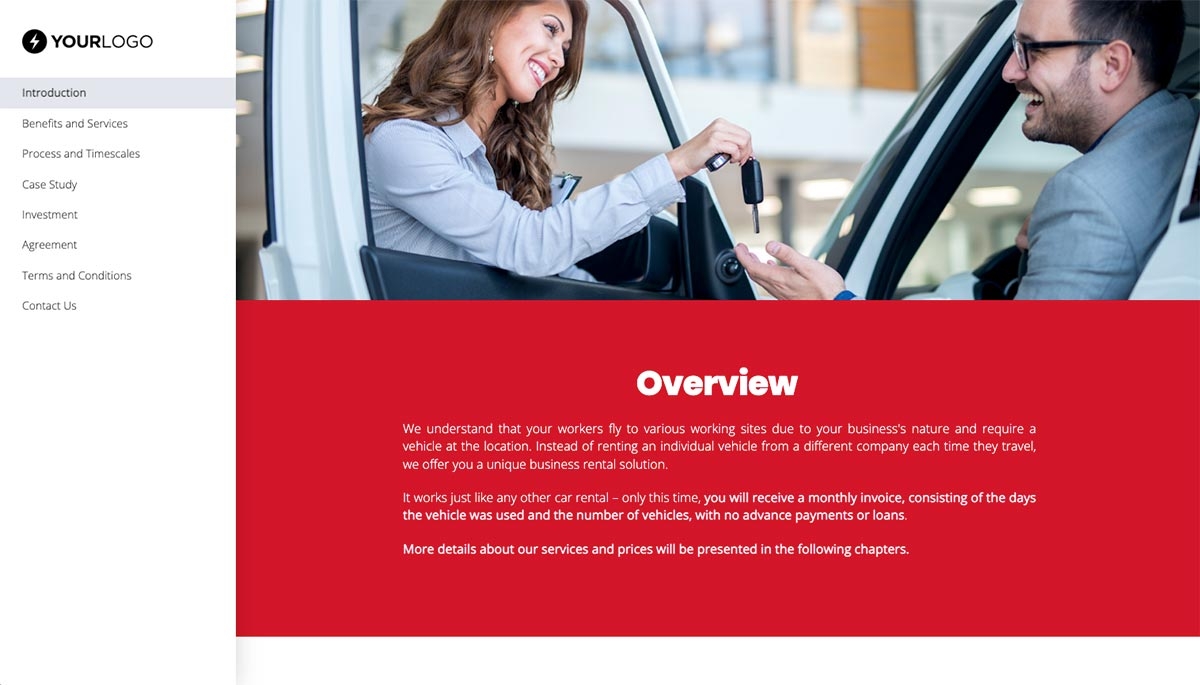This screenshot captures a website layout showcasing various sections aiming to present a business's service offerings. On the left-hand side, there's a vertical menu set against a clean white background, featuring black and gray text for easy readability. The menu, titled "Your Logo" at the top, includes the following options: Introduction, Benefits and Services, Process and Timescales, Case Study, Investment, Agreement, Terms and Conditions, and Contact Us. The 'Introduction' section is currently selected, highlighted against a gray-black background backdrop.

The main body of the website is split into two key areas. At the top, there is a vibrant photograph showing a candid moment between a man and a woman. The man, seated in the driver's seat of a white car with its door open, is receiving a set of car keys from the woman standing outside, leaning through the window. Both individuals share warm smiles, suggesting a positive and friendly interaction indicative of good customer service.

Below the photograph, a striking red background with white text features a compelling overview of the company's services. The text reads: "Overview: We understand that your workers fly to various working sites due to your business's nature and require a vehicle at the location. Instead of renting an individual vehicle from a different company each time they travel, we offer you a unique business rental solution. It works just like any other car rental, only at this time, you will receive a monthly invoice consisting of the days the vehicle was used and the number of vehicles, with no advance payments or loans. More details about our services and prices will be presented in the following chapters."

This descriptive caption provides a comprehensive understanding of the website's appearance and the contextual relevance of its various elements.